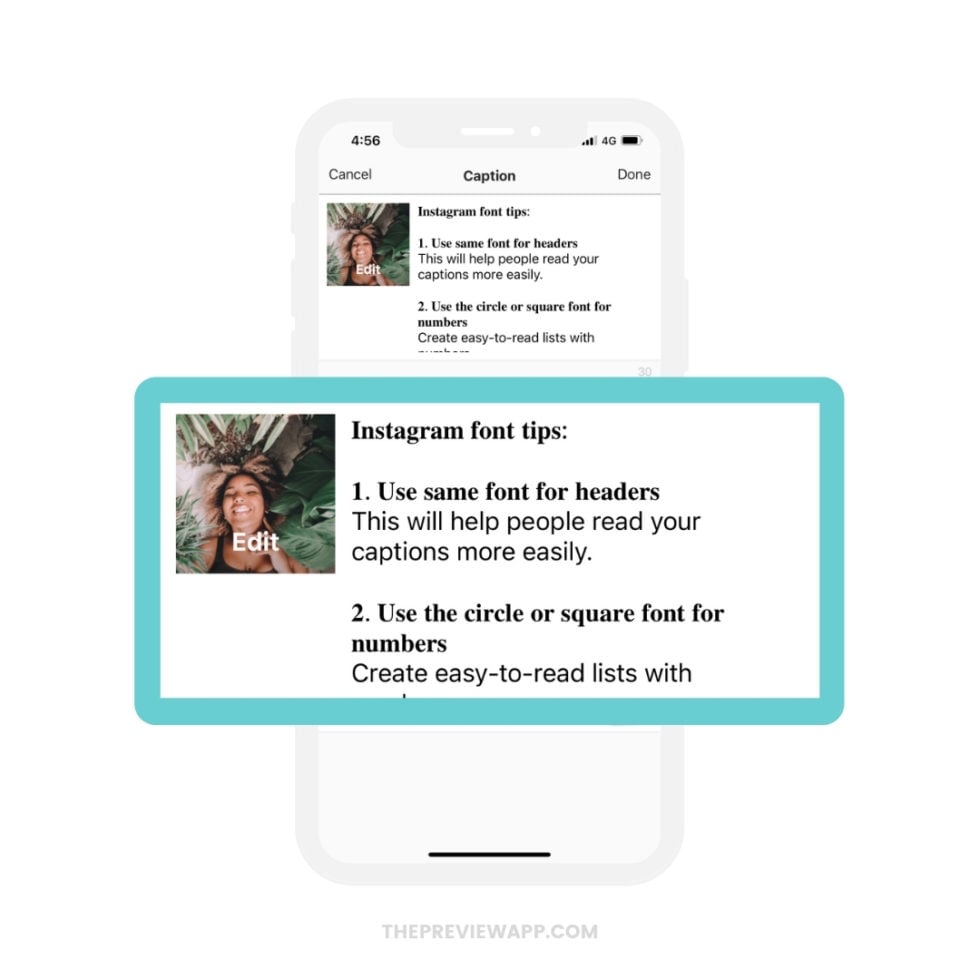**Screenshot Description: Instagram Font Tips Guide**

The image is a screenshot of a webpage that resembles an Instagram tip guide. At the center of the image, there is a semi-transparent white phone with a white background surrounding it.

- **Phone Details**:
  - **Top left corner**: Displays the time as 4:56.
  - **Top right corner**: Shows the phone's battery, which is almost full, the 4G signal, and notification symbols.

- **Content on the Phone**:
  - At the center, the phone screen shows text with tips related to Instagram font usage.
  - The title at the top reads: "Instagram Font Tips."
  - Below the title, there are two tips:
    - **Tip 1**: "Use the same font for headers. This will help people read your captions more easily."
    - **Tip 2**: "Use the circle or square font for numbers. Create easy-to-read lists with..." (The text cuts off here.)

- **Highlighted Area**:
  - The tips are presented within a light green, light blue, or turquoise-colored box.
  - In the top left of the box, there is an example font used for the tips, adding a practical illustration of the advice given.

Overall, the image provides a visually clean and well-organized guide to improving text readability on Instagram, though part of the content is cut off.